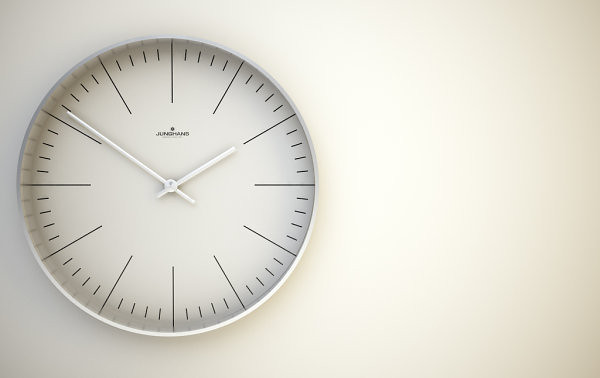The image features a minimalist clock mounted on an unadorned, cream-colored wall. The clock itself is also a subtle blend of cream and white hues, seamlessly blending with the background. Its design is simplistic yet elegant, with black lines in place of numbers, requiring one to intuitively gauge the time. The clock's edge is adorned with a delicate white-silver trim that mirrors the same tone as the slender hands ticking away inside. Though the brand name is visible, it's exceedingly small and indistinct. The clock displays a time of approximately 1:51. Notably, it is positioned off-center, leaning toward the left side of the wall, adding an asymmetrical balance to the composition.